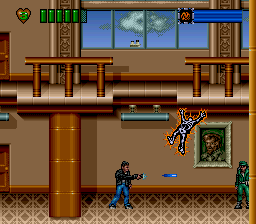In the on-screen gameplay image, a dynamic battle scene unfolds. At the bottom of the screen, a character aims a firearm emitting a vivid blue flame at another character clad in green, positioned on the opposite side. Above this intense firefight, a white, electrocuted character outlined in bright orange is depicted falling downwards, adding a chaotic element to the visual. The game's environment features a prominent brown pole supporting an upper level, giving a sense of structure to the scene. At the top of the screen, a user interface displays critical in-game information: a row of five green canisters representing lives and a heart-shaped brown icon bearing the number three, likely indicating remaining health points or lives. The intricate details and vibrant colors capture the fast-paced action and complexity of the game.